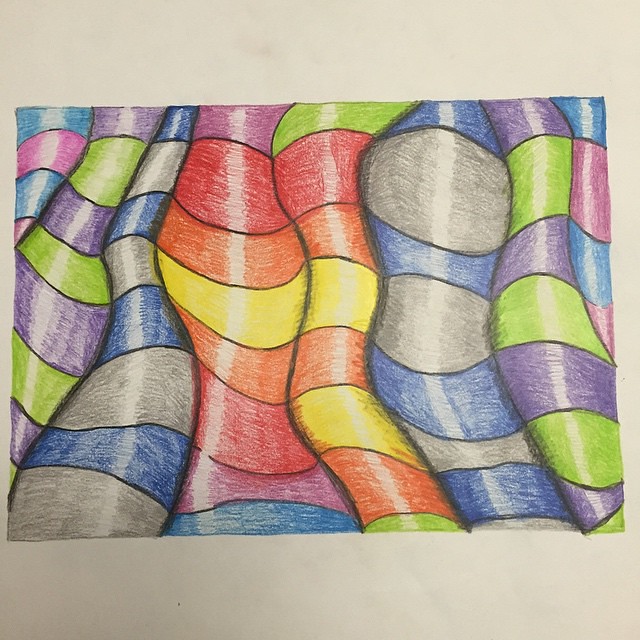A vibrant and detailed pencil drawing is showcased on a light gray background. The artwork depicts an array of vividly colored fabric folds that appear shiny, as if light is reflecting off them. The composition is organized in horizontal stripes with an intricate mix of colors. To the left, there are rows of folds in varying shades of purple and green. These stripes are followed by alternating folds in gray and blue. Adjacent to this, a band of multifaceted colors emerges, featuring red, orange, yellow, purple, and blue. Continuing towards the right, another section displays folds in a sequence of red, orange, and yellow hues. Finally, the drawing concludes with additional gray and blue stripes, leading back to folds in green and purple. The overall effect is one of luminosity and depth, capturing the dynamic and reflective qualities of fabric.